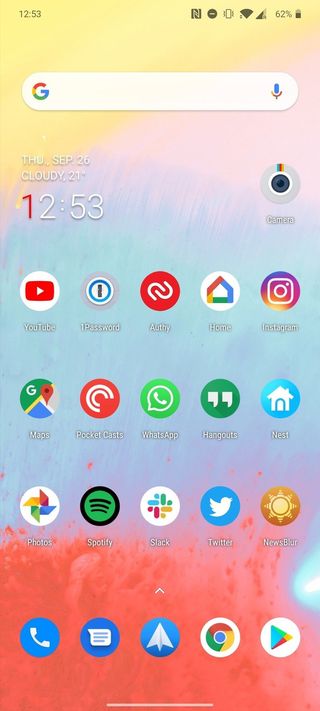Screenshot of a smartphone home screen taken at 12:53 PM. At the top left corner, the current time '12:53' is displayed, followed by a Google search bar just below. The date 'Thursday, September 26th' is shown along with the weather information, indicating 'Cloudy, 21 degrees'. The time '12:53' is repeated below the search bar.

Visible apps on the home screen include:
- YouTube
- WhatsApp
- Hangouts
- Twitter
- Slack
- Spotify
- Home
- 1Password
- Instagram
- Nest
- Photos
- Pocket Casts
- Chrome

Additionally, a row at the bottom features quick-access icons for the Camera, Messages, Phone, and Google Play apps. The arrangement and variety of apps suggest a well-organized and frequently used home screen setup, reflecting a blend of productivity, social media, and entertainment tools.